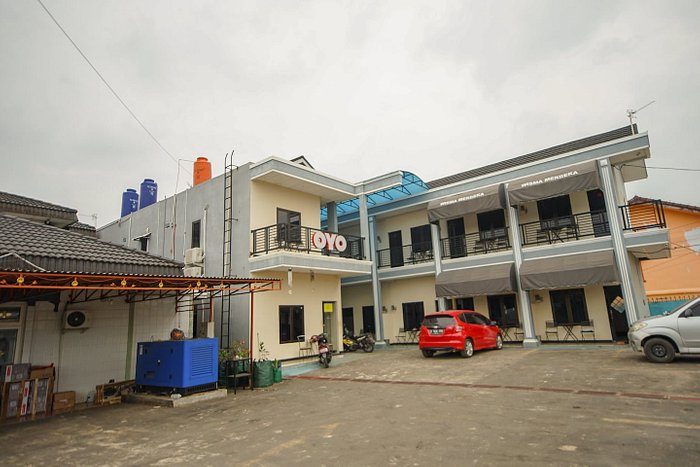The image depicts a modest hotel or motel, likely belonging to the OYO chain, characterized by its simple and functional design. Three distinct buildings are visible. The leftmost structure is a white, one-story building with a blue air conditioning compressor unit at the back and carton stock stacked by a back door, hinting at possible commercial usage. Next to it, a two-story white building features a balcony on the second floor with blue and orange chimneys and the "OYO" letters displayed prominently. A couple of motorbikes are parked in front of this building. The main hotel, adjacent to this, also has two stories and an uncovered, blue balcony running partially along the top floor. Visible are about seven rooms, each with a black door, double windows, and two black chairs outside. The hotel's name is on the awning above the second-floor rooms, though it's not completely legible. A red small SUV is parked in front of one of the rooms, alongside the front of a gray car partially visible on the right side of the image. The driveway and parking lot are concrete, with a slightly cloudy yet mostly sunny sky overhead. No greenery is in sight.